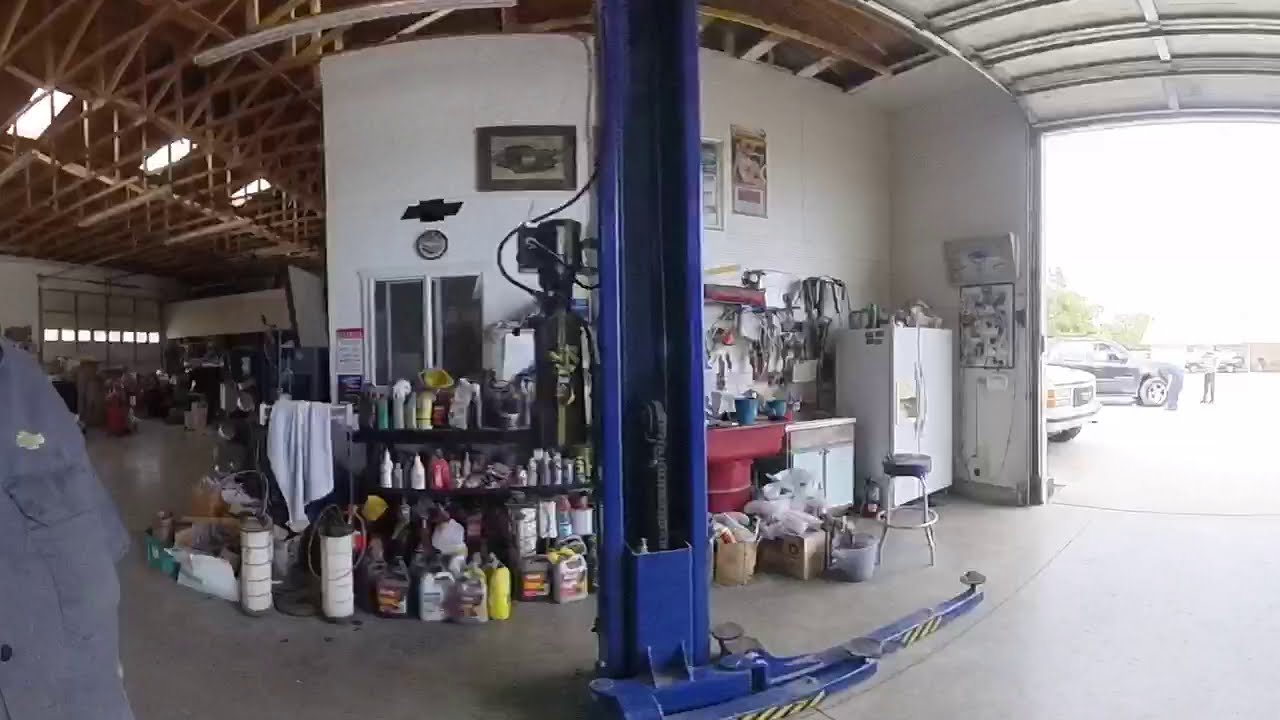In the fisheye view of a bustling auto shop, the lens distorts the vibrant scene, making everything appear slightly bent. Dominating the center is a prominent purple car lift, extending top to bottom with a black line running through its middle. On the lower right, a yellow and black caution-painted arm juts out. The eye is drawn to a backdrop featuring a white wall adorned with a black Chevrolet emblem. To the left, large windows with double frames illuminate shelves crammed with various spray bottles and containers, likely antifreeze or oil. Above, the unfinished wooden rafters of the roof are interspersed with skylights bringing in natural light. 

A refrigerator and a stool are nestled on the right side, alongside an outdoor sink cluttered with items hanging above it. The wide, light-gray concrete floor is split by a prominent crack that runs towards the left. An office area, characterized by sheetrock walls, a sliding window below a clock, and the Chevrolet logo above, sits prominently in the middle of the shop. 

On the far right, an open bay door reveals two people inspecting a black vehicle while the bright, glaring light from outside filters in. Parts of another lighter-colored vehicle are also visible outside. Additionally, the left side displays another bay area and a partially visible individual in a blue button-up shirt, adding a human touch to the mechanical ambiance. Despite a jumble of tools and boxes scattered around, the shop stands ready, waiting for the next vehicle to drive in.